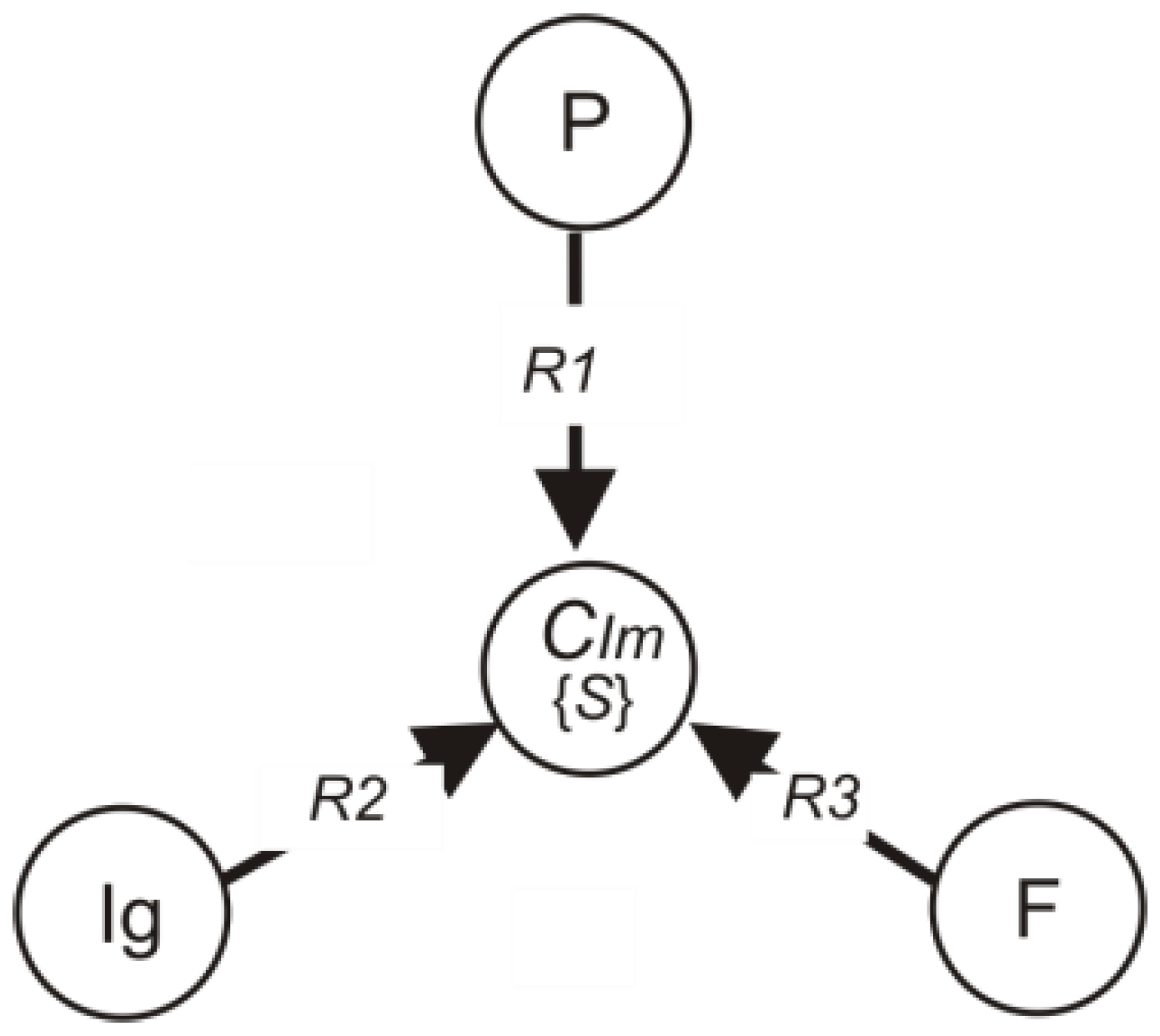The infographic illustrates a process flow, resembling a Y-shape, utilizing a series of labeled arrows and circles in black and white. At the top is a circle with a bold letter "P" inside, from which an arrow labeled "R1" descends toward a central circle. This central circle contains "CLM" with an "S" in brackets. To the left of the central circle is another circle labeled "LG," connected by an arrow marked "R2." On the right side, there’s a circle with the letter "F," and an arrow labeled "R3" also points towards the center. Each element is interconnected, depicting a clear flow ending in the central "CLM (S)" circle.